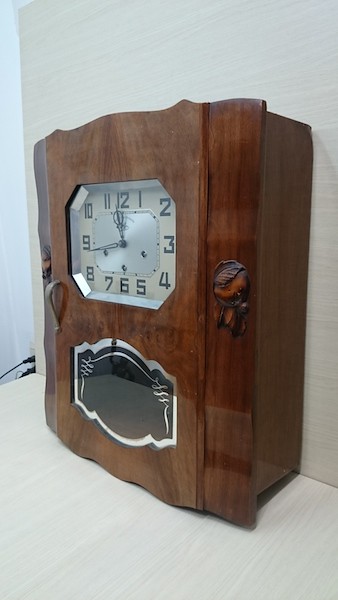This image showcases an old-fashioned clock residing on a gray-panel table against a gray-panel wall. The clock is enclosed in a medium, darker brown, shiny wooden casing with simple engraved designs and a beveled edge, adding to its vintage charm. The clock face is off-white with black numbers ranging from 12 to 11, surrounded by a brushed chrome or silver edge. Positioned at a noticeable 45-degree angle to the left, the clock features a distinctive diamond or gem-shaped face, with a matching black, shiny glass opening beneath, edged in silver. The clock reads a quarter to 12, and the front door—complete with a little handle—appears to open, though its purpose is uncertain. The scene includes visible power cords to the immediate left, hinting at other electronic devices nearby. Overall, the photograph captures the intriguing details of this ornate yet simple vintage clock, sitting elegantly against its muted background.